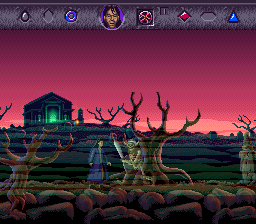The image is a pixelated screenshot from the Super Nintendo game "Warlock." At the top of the image, there is a light gray bar containing various icons: a red diamond, a blue triangle, a missing gem slot, a donut-shaped icon, a diamond-shaped icon, and a circular emblem featuring a red stick figure. In the center of this bar is a portrait of an old man with long black hair, dressed in a purple shirt, resembling a burnt Severus Snape. The main scene is set in a creepy, eerie forest with a crypt-like background illuminated by eerie green lights and a reddish sky. Dominating the center of the image is a sinister, wizard-like figure in a large, leafless tree, holding a sword. To the left of this central character stands another figure with long black hair and a blue robe. The terrain features dead trees, rocky textures, and a foggy, layered overlay indicative of the Super Nintendo's graphical capabilities. Also in the background, there's a house lit ominously with green light, contributing to the overall spooky atmosphere.